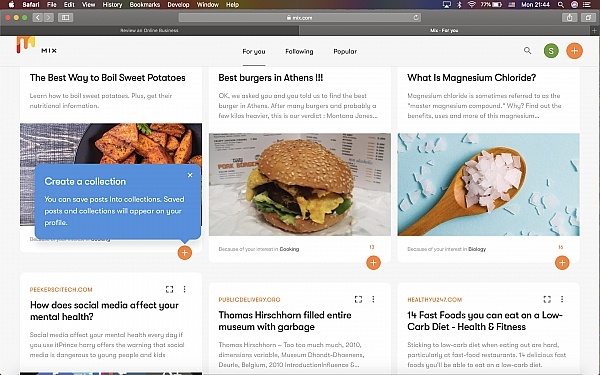This is a screenshot taken from Safari on an Apple device. The image prominently features the Apple logo at the top, followed by the word "Bafari" (likely a mispronunciation of Safari) written as "b-a-f-a-r-a-i". The menu bar displays options including File, Edit, View, History, Bookmarks, Develop, Window, and Help. 

On the right side of the menu bar, there is an icon indicating Bluetooth is on, the language is set to English, and the battery life shows 77%. Below the menu bar, the taskbar shows a blurred current website URL. 

The main content area appears to be a screenshot from a food-related blog or recipe website. The layout features an orange and yellow paint-like design with several clickable sections such as "For You," "Following," and "Popular." The "For You" section is active, displaying various articles. 

Among the highlighted articles are: 
1. "The Best Way to Boil Sweet Potatoes," accompanied by an image of boiled potatoes.
2. "The Best Burgers in Athens."
3. "What is Magnesium Chloride?" 
4. "How Does Social Media Affect Your Mental Health?"
5. "Thomas Hirschhorn Filled the Entire Museum with Garbage."
6. "Fourteen Fast Foods You Can Eat on a Low Carb Diet."

Each article has an option to save to a collection via a plus button at the bottom right of each content box. The top right corner of the page includes a magnifying glass icon for searching the site. The user is currently logged in to this website.